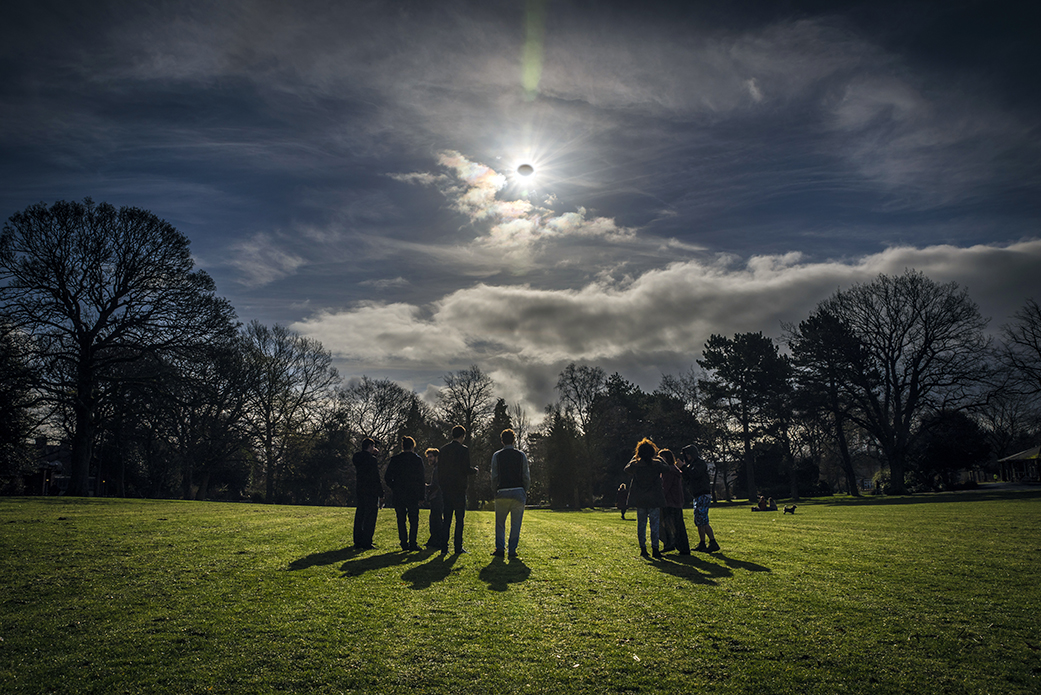The photograph captures a midsize group of people gathered in a green, grassy field, intently watching a solar eclipse. The event appears to be halfway through, with the moon partially covering the sun, positioned around the 10 o'clock spot in a dimming, cloudy sky. The image showcases enhanced contrast and altered color levels, giving it a distinctive visual tone. Wispy clouds partly obscure the sun, contributing to the overall darkened ambiance. In the background, a line of mostly leafless trees borders the horizon. Approximately nine people, primarily white, stand with their backs to the camera, gazing upwards at the celestial phenomenon. Shadows cast behind them suggest the time is either late afternoon or early evening. There also seems to be another group of spectators seated on the grass to one side.